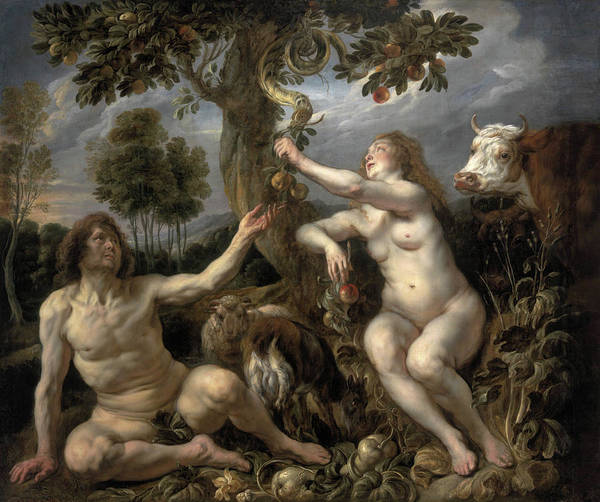This detailed painting artistically captures a biblical scene, likely representing Adam and Eve, in a Renaissance or 16th-17th century style. At the center of the image, the nude figures of Adam and Eve sit beneath an apple tree. Eve, positioned to the right, holds an apple in one hand while reaching up to grasp a branch with the other. Adam, kneeling beside her, extends his hand to pick another fruit. Both figures emit a subtle light that contrasts with the painting's overall dark tones, highlighting their forms against the muted earth tones of the setting. 

Surrounding them are various elements that add depth to the scene: a brown and white cow stands behind Eve, while several sheep lie around Adam on the ground. Gourd vines with large leaves grow at their feet, with one leaf strategically covering Adam's private area. In the distance, trees recede into the background under a sky filled with clouds, where a hint of moonlight or sunlight breaks through. The image distinctly lacks text, focusing solely on the visual narrative conveyed through a palette of green, gray, tan, yellow, orange, white, and red hues. The realistic and voluptuous depiction of the figures suggests a powerful allegorical representation of the well-known tale of temptation and innocence in the Garden of Eden.